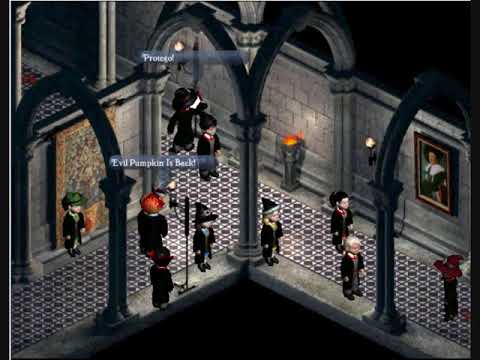In this image, we see a detailed screenshot from a video game, likely geared toward children, with an isometric viewpoint. The setting appears to be inside a castle, characterized by gray stone brick walls. At the bottom left of the screen is an entryway. The scene features intersecting walkways that run diagonally from the bottom right to the upper left and another from the bottom left to the right. Stone pillar archways line the hallways, some with flame torches.

The central focus of the image includes several animated characters, reminiscent of Lego figures, dressed in outfits that suggest a magical theme—some wearing pointy wizard hats and black cloaks, similar to characters from Harry Potter. These characters stand together in the center of the screen, almost soldier-like in their stillness. 

On the walls, particularly the bottom right, various pieces of artwork, including portraits, are displayed. Lit candles and a patterned carpet add to the detailed castle interior. Prominent text on the image announces, "Evil Pumpkin is Back" and "Protego," hinting at a storyline or mission within the game. The primary color palette includes shades of gray, orange, green, black, white, and tan, creating a vivid and immersive environment.